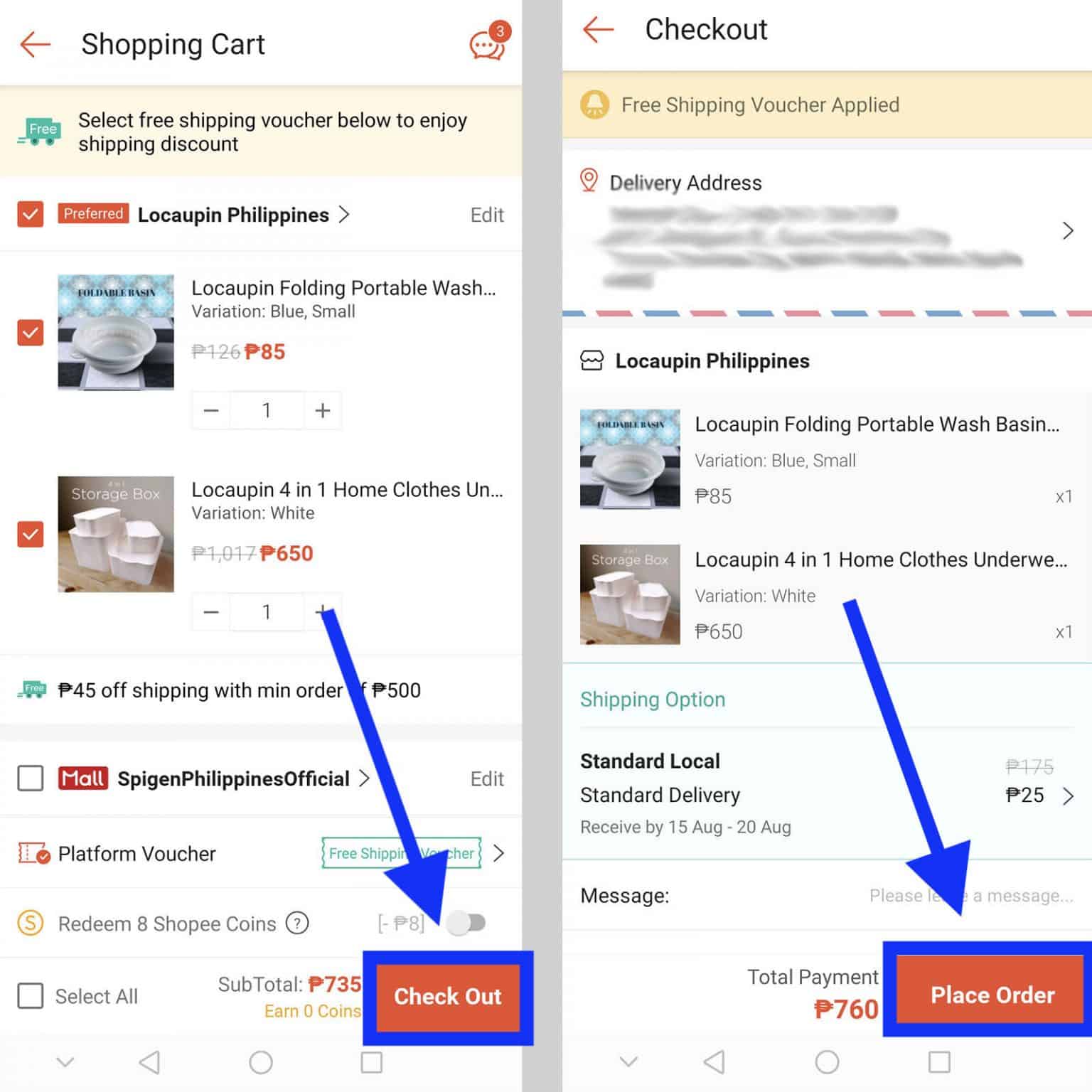**Detailed Image Caption:**

*Left Side: Online Checkout Interface*

The left side of the image features an online checkout interface from a Filipino e-commerce platform.

- **Top Section**:
  - The top left corner displays the text "Shopping Cart" in bold black letters, accompanied by an orange left-facing arrow.
  - Adjacent to it on the right, there is a red speech bubble icon with three white dots and a red circle containing the number "3."
  - Below these, there is a peach-colored banner with a green truck icon and the word "FREE" in white letters. This banner reads, "Select free shipping voucher below to enjoy a shipping discount," in both black and white text.

- **Main Area**:
  - A white box with an orange square and a white check mark is visible, and next to it, a long orange bar reads "Preferred and Signed" in white letters.
  - The text "Luca penned the Philippines" appears with a gray sideways V and the word "Edit" in gray on the far right.

- **Product Listings**:
  1. **First Product**:
     - A small image of a white bowl with black text on a blue banner is shown.
     - The description to the right reads, "Volca pens, folding, portable, wash...", with the variant as "blue, small."
     - The original price is struck through (₱126), and the discounted price (₱85) is displayed in orange.
     - Below is a quantity adjustment box showing the number "1."

  2. **Second Product**:
     - An image depicts several white boxes stacked on a wooden counter with a gray background.
     - The right-side text reads, "Loca pen, 4 in 1, home clothes, UN..." with the variant "white."
     - The original price (₱1017) is struck through with the discounted price (₱650) highlighted in orange.
     - Again, a quantity box with the number "1" is shown.

- **Bottom Section**:
  - A blue arrow points towards a blue-rimmed box with an orange check mark inside and the text "Checkout" in white.
  - Below this, the text "₱45 off shipping with min order ₱500" is displayed alongside the free truck icon.
  - To the right, a checkbox with a red square contains the text "Mall," and next to it, "Big in Philippines Official" can be seen with a gray V and the word "Edit."
  - Separated by a gray bar, there is a "Platform Voucher" icon with a red circle and white check mark.
  - Further down, an aqua-rimmed box with the text "Free Shipping Voucher" is slightly overlaid by the blue arrow.
  - Another section reads, "Redeem Shopee Coupons" in black, with a gray circle and a minus “P8” discount visible.
  - At the very bottom, "Select All" and "Subtotal: ₱7535" are shown, followed by the text "Earned 0 Coins" in orange.

*Right Side: Checkout Summary*

The right side showcases a similar online checkout summary.

- **Top Section**:
  - The text "Checkout" features a left-facing orange arrow.
  - A peach-colored section displays an orange bell icon with "Free Shipping Voucher Applied" in black text.
  - Below, the delivery address is indicated with a red location icon (details are redacted).

- **Main Area**:
  - The same two product images and descriptions appear, but with no original prices crossed out, only the current prices displayed.
  - Additionally, next to both products, the quantity "x1" is shown.

- **Shipping Options**:
  - A green header reads "Shipping Option."
  - Listed below are "Standard Local" and "Standard Delivery" options with the price of ₱175 crossed out and ₱25 marked in blue.
  - Delivery dates are specified as "15 Aug - 20 Aug."

- **Bottom Section**:
  - The word "Message" appears in black, with the placeholder text "Please leave a message" in faint gray.
  - The total payment amount is displayed as ₱760 in orange.
  - A blue arrow points to a "Place Order" box, rimmed in blue and orange with white text.
  - The usual navigation buttons are positioned at the very bottom.

These two sections are divided by a long gray bar running vertically between them.